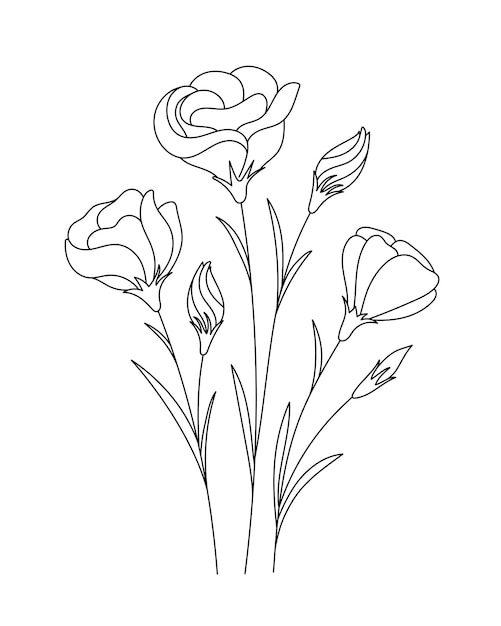The image is a hand-drawn, black line illustration of three long-stemmed flowers reminiscent of rosebuds. Each flower stem features a fully bloomed flower at the top and a smaller bud adjacent to it. The illustration is minimalistic, utilizing thin, black outlines against a stark white background, creating a clean and simple aesthetic. The flowers have tightly clustered petals, long stems, and sparse, elongated leaves. Notably, the central stem has a split, forming two branches, each with its own combination of a fully bloomed flower on the left and a bud on the right. The buds appear to be in various stages of development, with one nearly 80% bloomed compared to the others.